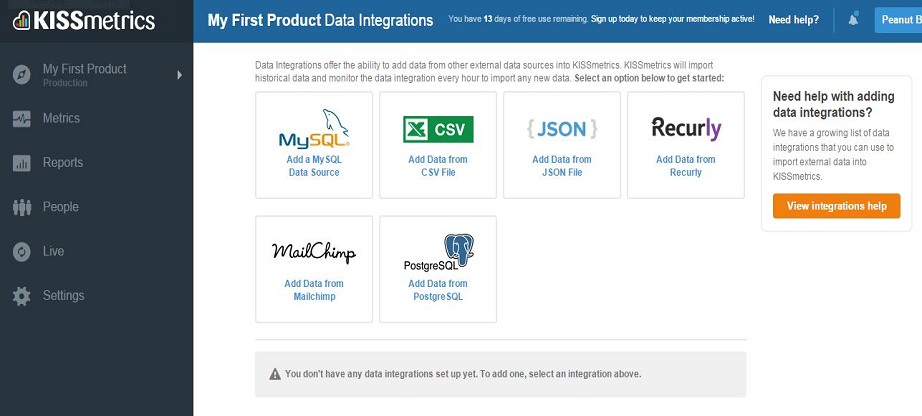A detailed description of a webpage captured in a photograph:

The image portrays a webpage with a blue banner at the top displaying the text "My First Product Data Integrations" in white. Below this banner, a message indicates, "You have 13 days of free use remaining. Sign up today to keep your membership alive," with a "Need Help?" button positioned to the right.

On the left side of the page, a heart icon tilted sideways, lined with red and green, appears with the text "KISS" in large white font and "metrics" in smaller white font beneath it. A black vertical panel adjacent to the heart icon lists navigation options: "My First Product," "Production," "Metrics," "Reports," "People," "Live," and "Settings."

The main section of the page features several square boxes, each representing a data source integration option. These options include:
- "MySQL": allowing the addition of a MySQL data source.
- "CSV": enabling the addition of data from a CSV file.
- "JSON": providing the option to add data from a JSON file.
- "Recurly": facilitating the addition of data from Recurly.
- "MailChimp": offering the option to integrate data from MailChimp.
- "PostgreSQL": allowing the addition of data from a PostgreSQL database.

Each integration option is visually distinguished by its label and purpose, contributing to the page's organized and user-friendly layout.